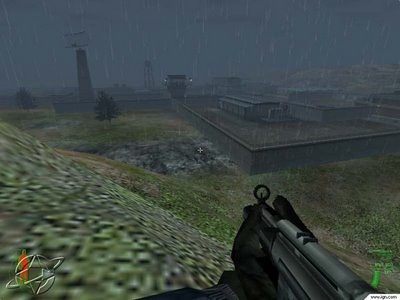The image is a color photograph, slightly blurred towards the background. Dominating the foreground is a detailed semi-automatic black gun. The photograph features a small, shady white icon near the front, resembling a globe encircled by a ring. On the right side of the image, there is a prominent green area. Along the bottom, there is small, illegible text. The background includes rolling hills, flat-roofed buildings layered with additional structures, and towering edifices interspersed with trees. The possibility that the image is computer-generated cannot be ruled out.